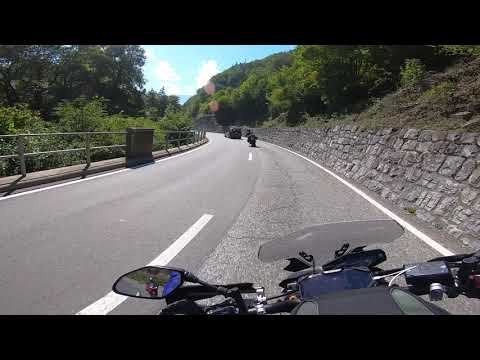This image is an exterior daylight photograph taken from the perspective of a person riding a black motorcycle on a two-lane paved road, framed by thick black letter bars on the top and bottom. The scene captures the handlebars, clutch, and left-side rearview mirror of the motorcycle. In the left-hand mirror, there's a reflection of another motorcyclist on a red motorcycle riding behind. The rider is in the right lane of the road, which is lined on the right by an angled gray stone wall at the base of a hill that ascends into a natural area filled with grass, trees, and shrubs. On the left side of the road, there's a metal guardrail beyond which the land drops sharply into a forested area. Ahead in the right lane, another motorcycle is visible, with a non-motorcycle vehicle, possibly a truck, further up the road. The road itself curves gently to the left under a bright blue sky, dotted with fluffy white clouds, capturing the serenity of an outdoor setting with minimal traffic.